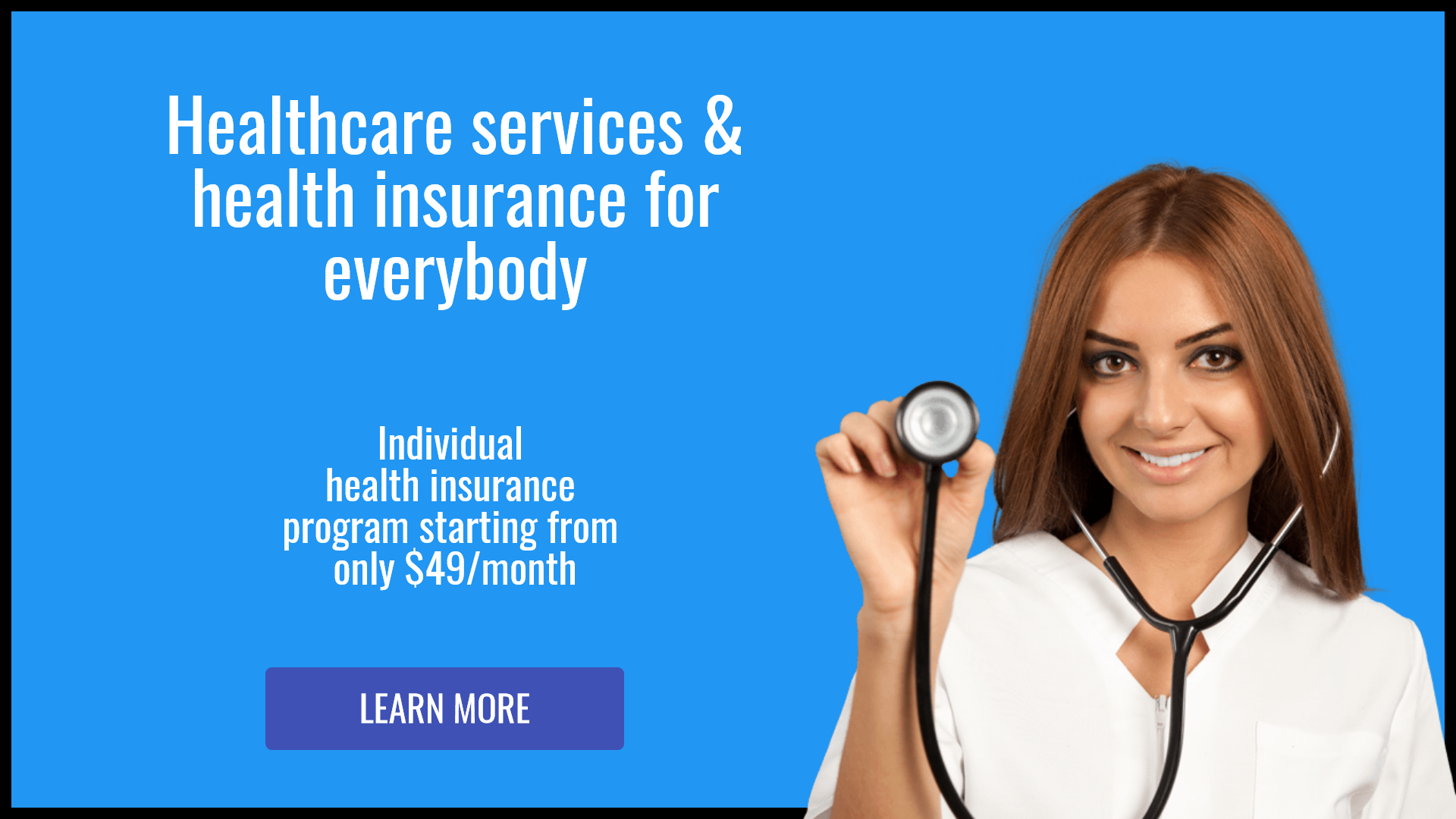**Caption:**

In this simple yet captivating healthcare advertisement, a young, attractive woman with long brown hair is featured prominently against a vibrant blue background. She listens intently through a stethoscope, with its heart-shaped end held up to the camera, as she beams with a warm and welcoming smile. Clad in a crisp white shirt, she exudes professionalism and approachability. The woman, who appears to be of Hispanic or Greek origin, adds a touch of diversity to the ad, though her exact background remains ambiguous.

To the left of the image, white text spans two-thirds of the space, declaring, "Health Care Services and Health Insurance for Everybody." It goes on to promote an individual health insurance program that starts at an affordable $49 per month. Below this message, a conspicuous purple button invites viewers to "Learn More," encouraging further engagement.

The overall design is framed with a black border, adding a touch of definition to the predominantly blue backdrop. Despite the clear and concise presentation, the advertisement does not specify the company or service provider offering this inclusive health care insurance.